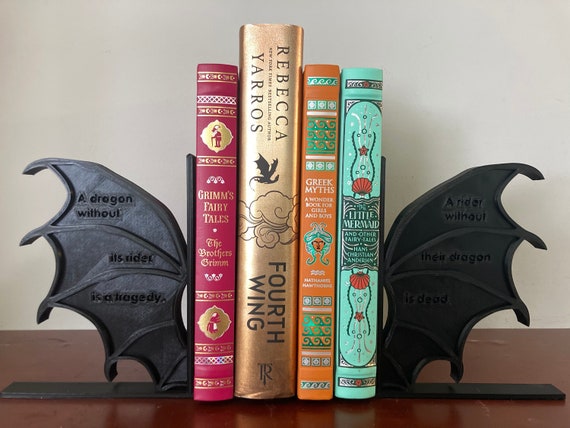The image features a collection of four books flanked by distinctive dragon wing bookends on a brown table. The bookends are black, resembling wrought iron, with the left one inscribed, "A dragon without its rider is a tragedy," and the right one displaying, "A rider without the dragon is dead." The books in between are "Grimm's Fairy Tales" in red, "Fourth Wing" by Rebecca Yarros in gold, "Greek Myths" in orange with green lettering, and "The Little Mermaid and Other Fairy Tales" by Hans Christian Andersen in teal. The backdrop is a simple tan or white wall, adding to the overall minimalist aesthetic of the scene.